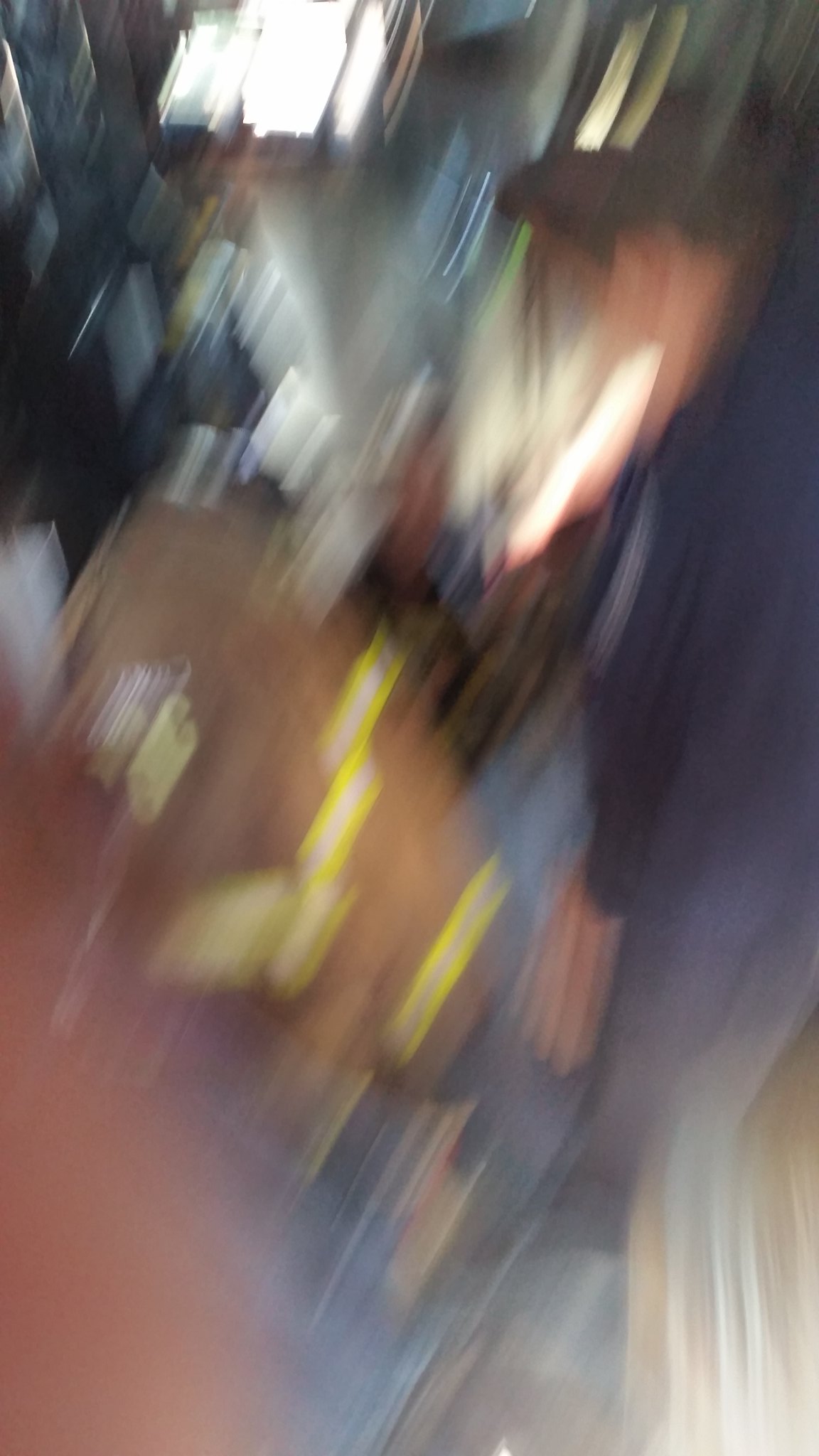The image depicts a highly blurred and fast-motion scene that appears to be taken indoors, possibly inside a hallway or corridor. Central to the image is a Caucasian man with brown hair, dressed in a dark sweatshirt and blue jeans, who is leaning slightly forward with his head tilted down. His hands are vaguely defined, possibly resting on or near a chair, adding to the impression of motion and intensity in the photo. Surrounding him are chaotic streaks and shapes in vibrant colors—yellow, red, blue, and green—likely caused by a long exposure or fast movement, creating an effect reminiscent of neon lights. The background features darker-colored walls, possibly gray or blue, and a floor that may be a gray carpet or a red surface, contributing to the confusing visual elements. At the top center of the image, a square window lets in a significant amount of daylight, which appears to add to the overall light distortion and blurriness. The bright natural light streaming in from the window exacerbates the surreal and almost alien atmosphere of the photograph. Overall, the entire scene is dominated by a sense of motion and indistinct forms, making it challenging to discern specific details.